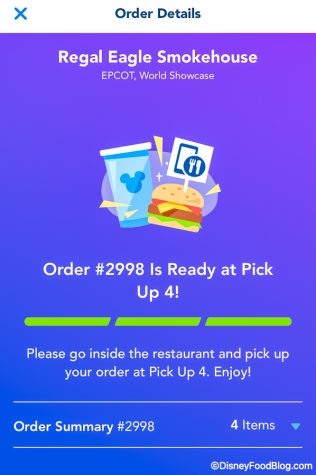The image is a detail-rich screenshot of an order confirmation from the Regal Eagle Smokehouse at Epcot, World Showcase. The top portion features a white navigation bar with a blue "X" located in the top left corner for closing the window, and "Order Details" displayed prominently in bold, blue text.

Below this header, a striking, royal blue vertical rectangle captures the viewer's attention. Within this rectangle, the text "Regal Eagle Smokehouse" is boldly printed in white at the top, followed by the location specification "Epcot, World Showcase."

The centerpiece is a charming, retro-styled Disney cartoon, showcasing a blue cup with a white lid, adorned with a blue Mickey Mouse silhouette. Beside it, an appetizing cheeseburger is illustrated, complete with a toothpick holding a sign that features icons of a smartphone and a fork and knife.

This visual segment is accompanied by the text "Order Number #2998," indicating that the order is ready for pickup at Station 4, emphasized by four exclamation points.

A thick, dashed lime green bar segments the image, adding to the visual hierarchy, followed by a directive to "Please go inside the restaurant and pick up your order at Pickup 4. Enjoy."

Further down, a thin white line separates the order summary, reiterating "Order Summary #2998" with "Four Items" indicated on the right-hand side. A blue downward-pointing arrow suggests that more details about these four items can be accessed.

The image concludes with another thin white line and the text "© DisneyFoodBlog.com" in the bottom right corner, crediting the source of this detailed and visually engaging order confirmation.